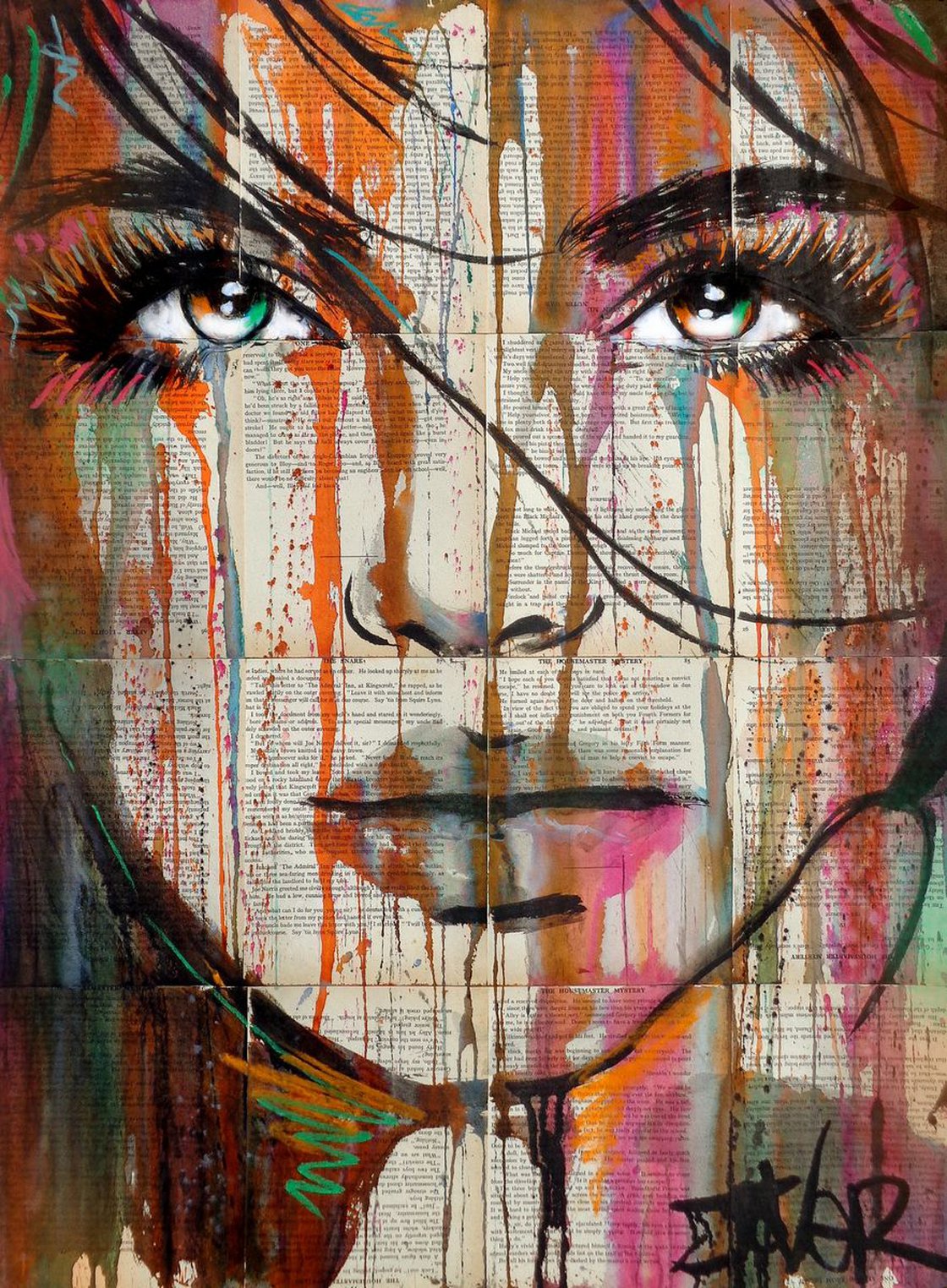This artistic painting features a highly detailed and evocative portrait of a woman. Rendered in a style reminiscent of comic book artistry, the face of the woman dominates the composition, occupying nearly 90% of the image. Her facial features are carefully crafted to appear attractive, with long eyelashes and defined eyebrows. The eyes, strikingly colored amidst the primarily black and white drawing, are a captivating mixture of green, white, and orange.

The woman's visage appears superimposed upon a collage of book pages, their yellowish-beige backgrounds and black text clearly visible, giving the painting a unique and layered texture. This choice of medium contributes to the artwork's intriguing blend of classical and contemporary elements.

Colors cascade over her monochromatic face in vibrant drips and splashes of orange, brown, purple, teal, and red, enhancing the dynamic composition with an impressionistic touch. The lips are highlighted with a blend of red, pink, brown, and black, adding to the overall vibrant aesthetic. Beneath her chin, additional colorful splashes bring further life and energy to the piece.

The artist's signature, "J-A-V-E-R," is inscribed in the bottom right-hand corner, adding a personalized stamp to this unique and visually compelling artwork.